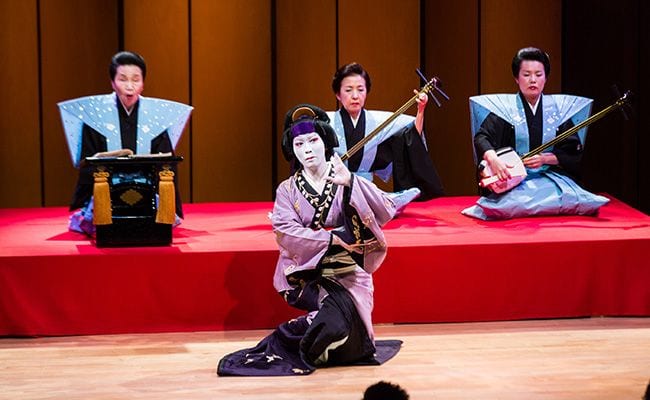The photograph depicts an oriental musical performance on a rectangular, horizontally oriented stage. Dominating the foreground is a dancer, dressed in a striking light purple satin outfit with dark violet accents, complete with flowing robes and painted white face and hands, reminiscent of a geisha or mime. Behind her, three musicians, adorned in traditional blue attire, are seated cross-legged on a red-carpeted platform. The first two musicians hold string instruments, similar to banjos, using their left hands to play the strings and their right hands to strum. The performer on the far left appears to be singing, possibly reading from an open book placed on a pedestal in front of her. The backdrop features a subdued, brown set wall, providing contrast to their colorful attire and the vibrancy of the red stage. This rich and culturally immersive scene captures the harmony of music and dance in a traditional setting.